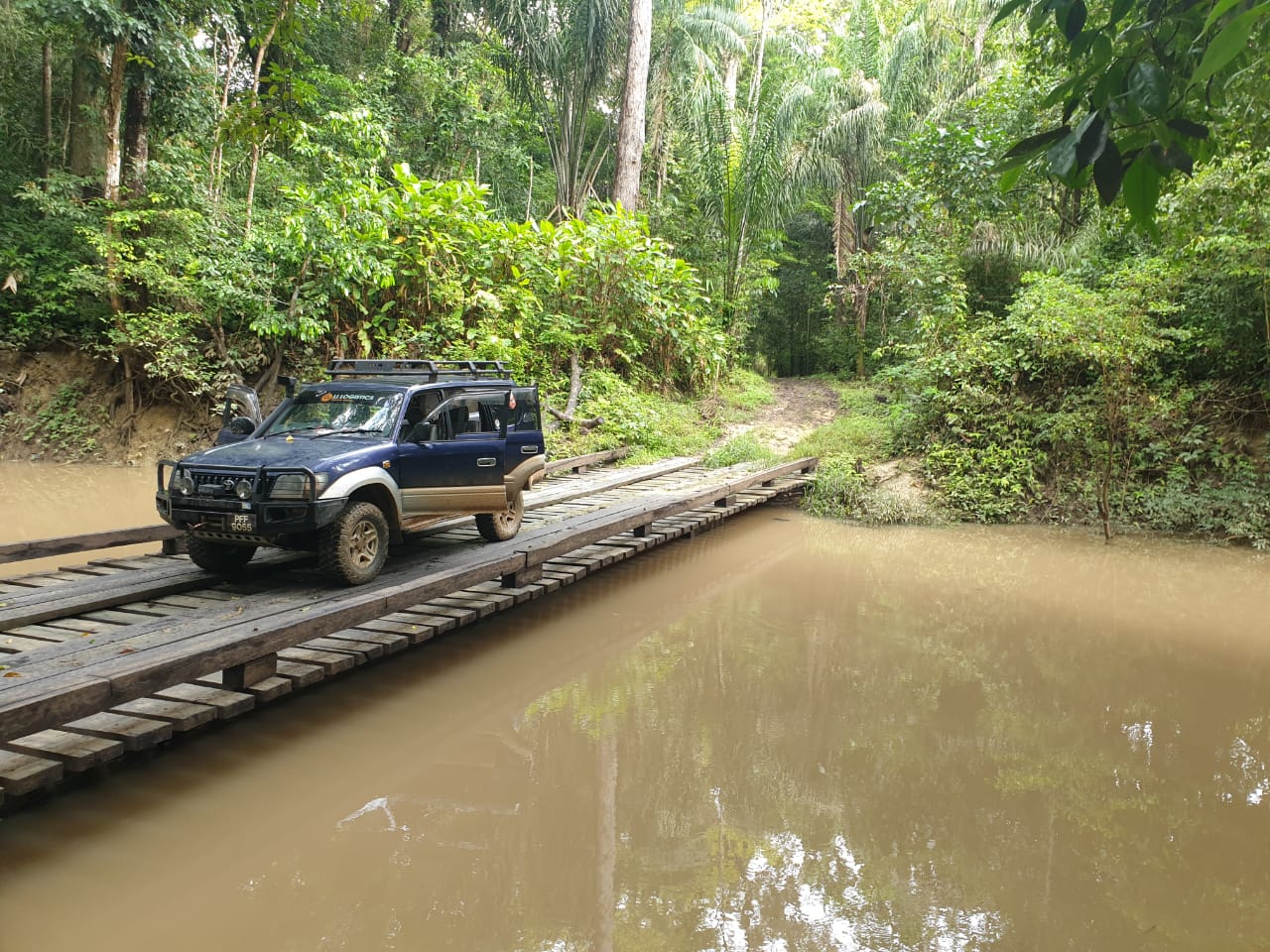In this vivid photograph, a two-tone blue and gold SUV, reminiscent of a Jeep Wagoneer, sits parked with all its doors wide open on a very narrow, wooden bridge. The bridge, constructed from wooden slats and equipped with a low railing, spans over murky, muddy, light brown water. This vehicle, which is a bit dirty and outfitted with metal brush guards and outcropping lights characteristic of safari-type vehicles, also features a large metal rack on top. The bridge only accommodates one car at a time. The scene is captured with great clarity, likely using a modern-day camera. The vehicle appears unmanned. Surrounding the bridge and stretching into the background is a dense tropical jungle, brimming with various types of trees, including palm trees, and an assortment of lush green shrubs and ground cover. A dirt path in the background blends into this verdant forest, suggesting a route deeper into the rainforest. This particular setting evokes a sense of adventure and a touch of mystery, with a stopped vehicle hinting at an untold story within this vibrant, natural environment.